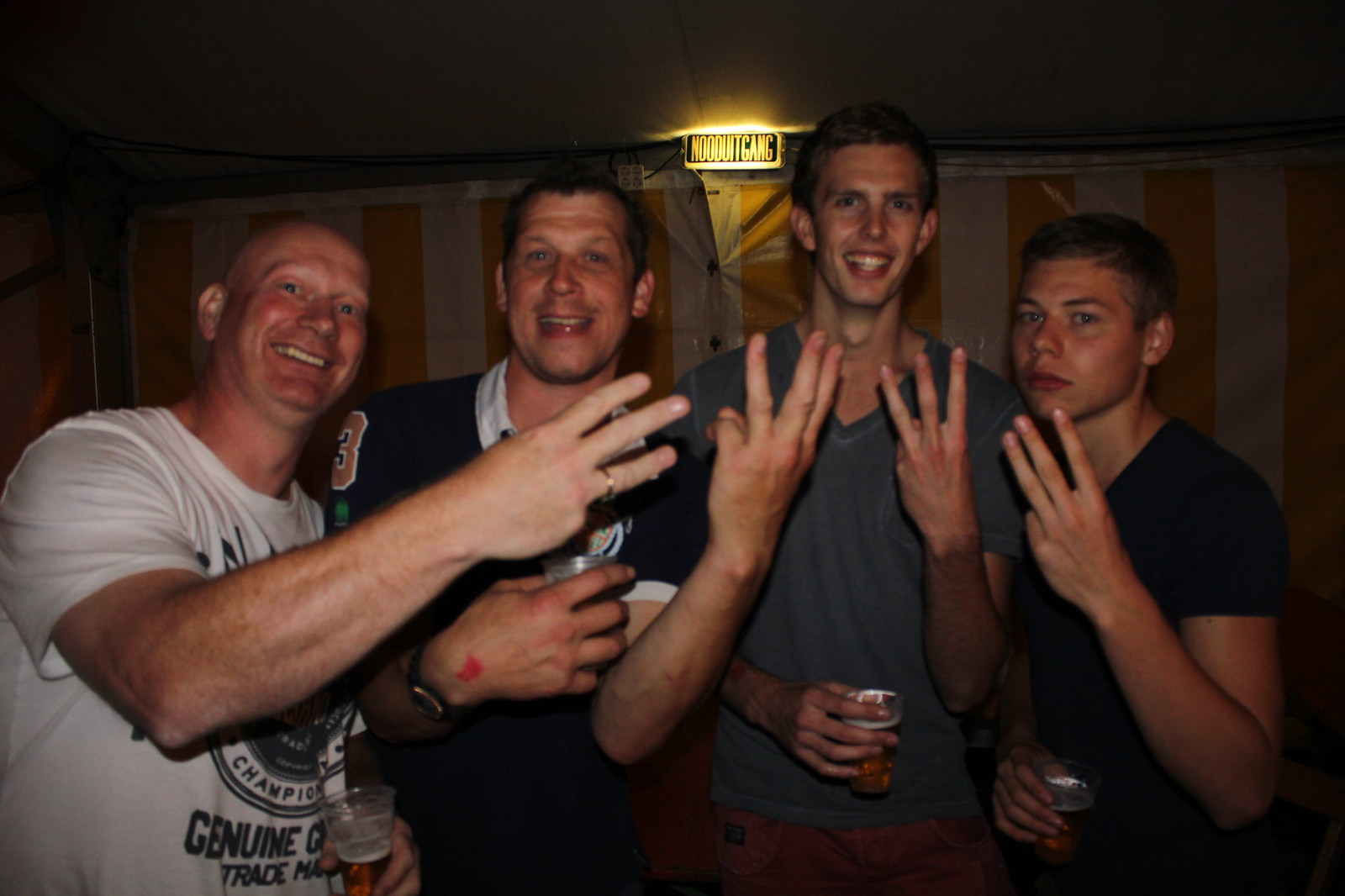The image depicts a joyful group of four men holding small plastic cups of beer, standing in front of a yellow and white striped tent. The tent is buttoned together in the middle. A glowing neon sign in the background, reading "No Do It Gang," adds a festive touch to the scene. The men, illuminated by flash photography in a dimly lit room, are all making a gesture with their left hands, extending three fingers.

Starting from the left, the first man is bald, wearing a white t-shirt with a green logo, and is smiling broadly. He proudly displays a wedding ring and extends three fingers with his left hand. Next to him stands a middle-aged man in a blue polo or rugby shirt with a white collar, mirroring the three-finger gesture with his left hand as well. The third man, who is the tallest, is dressed in a gray v-neck shirt and red shorts. He too holds his beer in his left hand while making the same three-finger sign. The final man on the far right, the shortest and appearing youngest, is wearing a navy blue v-neck shirt. Unlike his companions, he carries a more serious expression but still participates in the shared gesture. The camaraderie among the men is evident despite the dim setting, and the entire scene is infused with a sense of unity and cheerfulness.